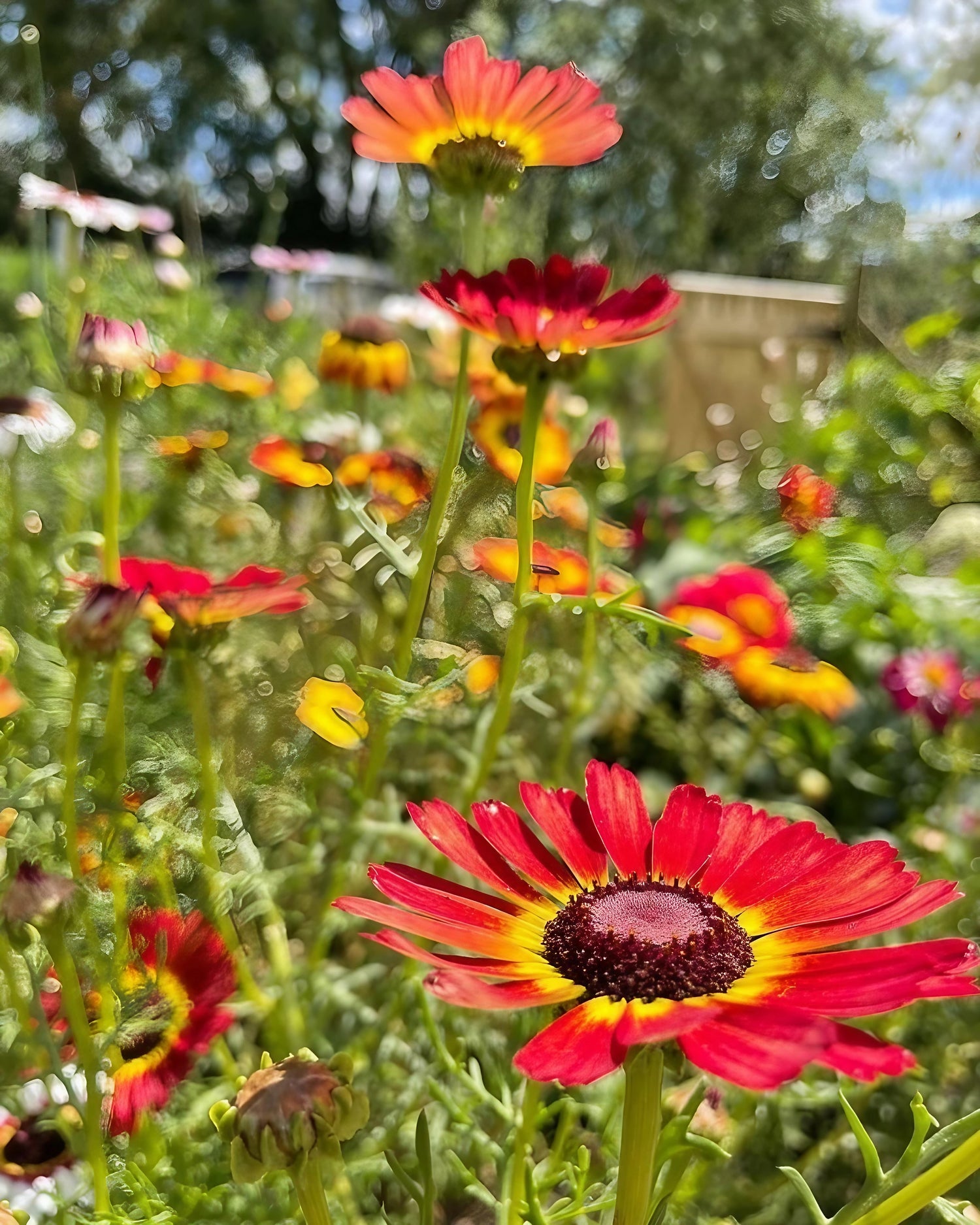The photograph captures a beautifully vibrant garden scene on a sunny day. At the forefront, a prominently defined poppy with strikingly narrow red petals stands out, transitioning to yellow at its center and enclosing a maroon to dark red core. The flower rests on a robust green stem and is surrounded by an array of over 20 similar blooms, though less detailed due to the image’s intentional blurriness. This creates an artistic effect, suggesting a natural meadow feel or perhaps an intimate backyard corner with hints of a fence or shed obscured by the focus. The flowers, resembling daisies or zinnias to some, rise to about 2 feet tall, embedded in lush green foliage. The background features an indistinct tree line and patches of blue sky, enhancing the serene and colorful atmosphere of the photo. Different stages of the blossoms—from partially closed to fully open—add depth to the scene, painting a picturesque, relaxing, and inviting garden landscape.